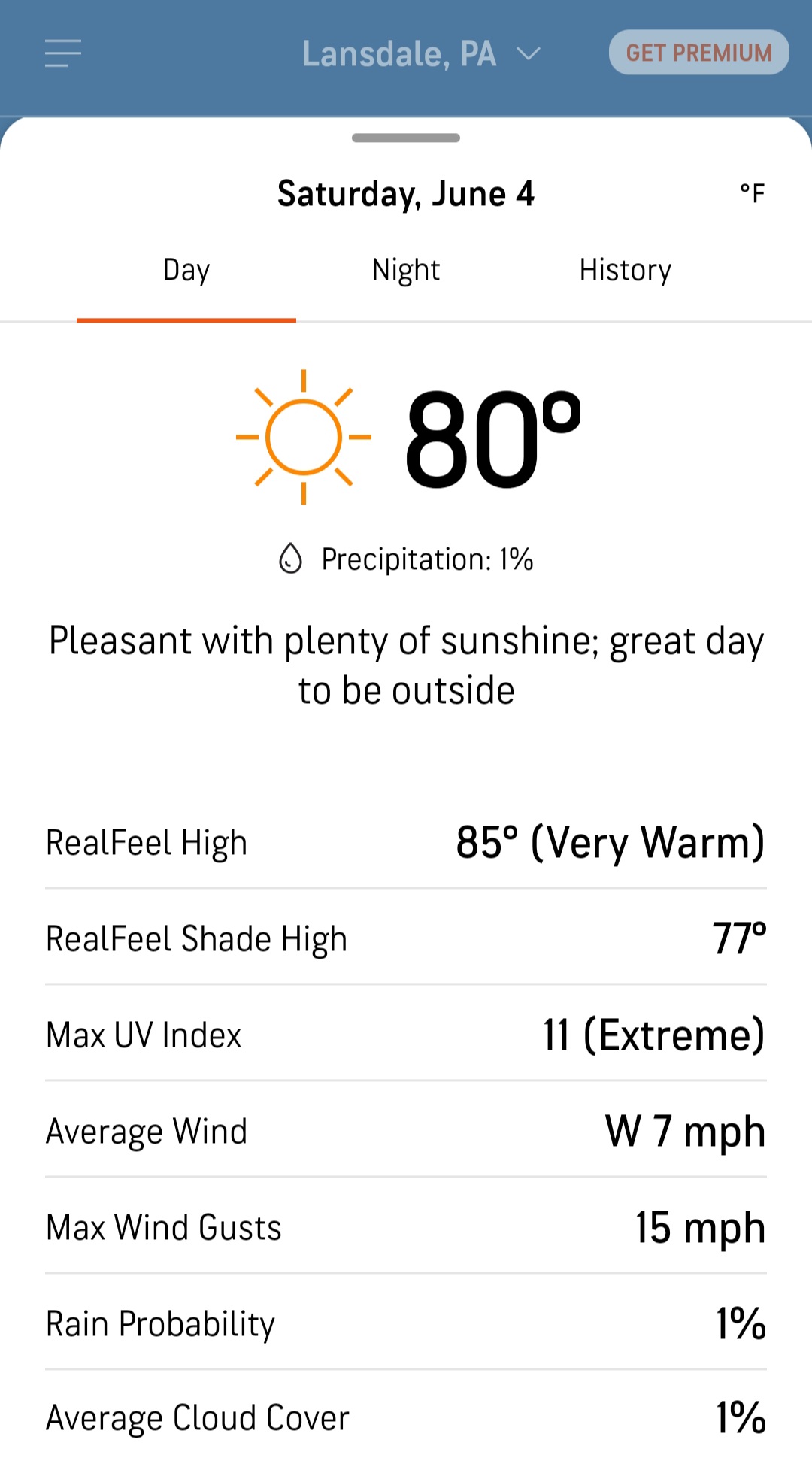**Screenshot from Weather App**

In the upper left corner, a blue banner is displayed, featuring a three-line menu icon. Centrally located on the banner, "Lansdale, PA" is shown alongside a drop-down arrow, while to the far right, an oval-shaped "Get Premium" button is present. Below this banner, a thin gray line stretches across the screen.

The date "Saturday, June 4th" is prominently bolded, with the Fahrenheit symbol to its right. Directly below, an orange-underscored "Day" tab is visible, flanked by options for "Night" and "History."

The weather details begin with a sun icon followed by "80°" in large, bold font, denoting the daytime high temperature. Below this, "Precipitation 1%" is indicated with a water droplet icon. Centered beneath, a summary reads, "Pleasant with plenty of sunshine. Great day to be outside."

Further information includes:
- RealFeel® High: [Data not specified]
- RealFeel® Shade High: 70°
- Max UV Index: 11 (Extreme)
- Average Wind: W at 7 MPH
- Max Wind Gusts: 15 MPH
- Rain Probability: 1%
- Average Cloud Cover: 1%